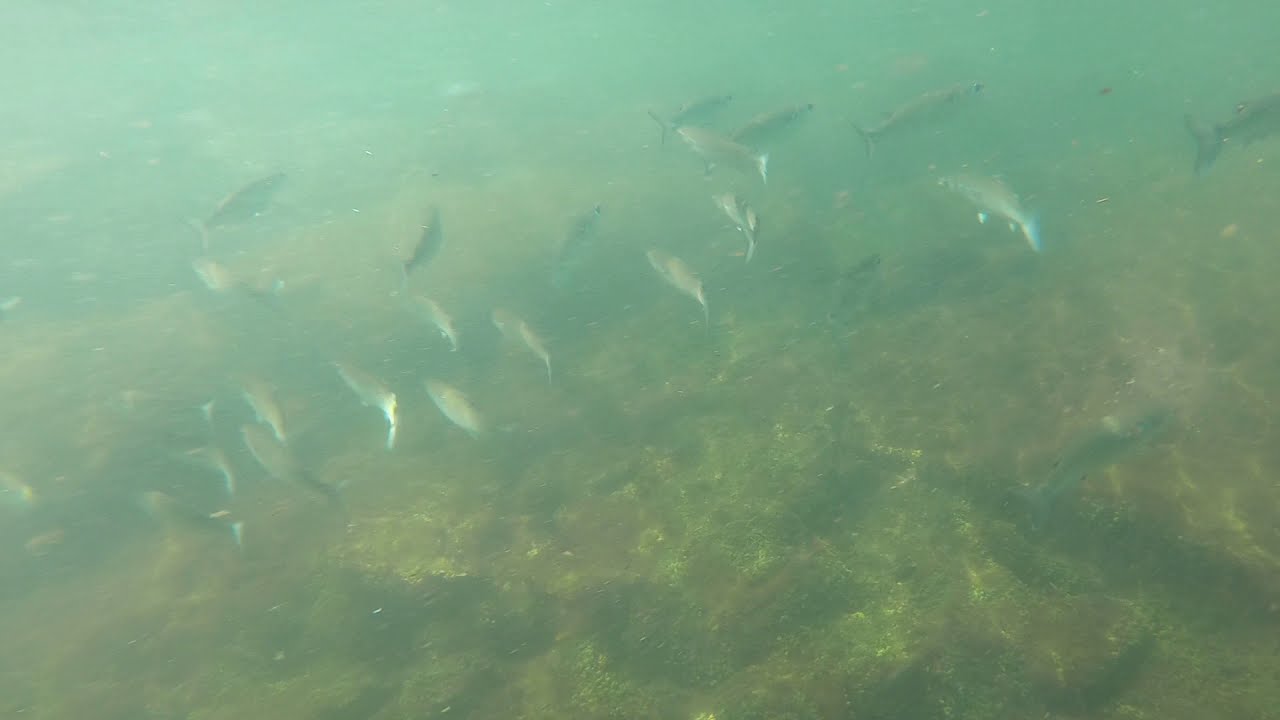This horizontally aligned rectangular image depicts an underwater scene of a greenish-gray tinted, somewhat murky body of water, aiming downwards. The focus is primarily on a dense concentration of fish, varying in size from smaller, silvery ones to larger, more grayish ones. Some fish are swimming towards the camera while others swim in the opposite direction, creating a dynamic sense of movement. Light from above casts reflections and shadows, enhancing the visibility of their fins and tail fins, though the image remains somewhat blurry. Below the swimming fish, the ocean floor is visible, revealing a mixture of grayish-white and green hues, with larger, darker grayish-brown rocks scattered across it. The upper portion of the image shows fewer fish and transitions into a more uniform greenish-gray color. There is no text in the image, keeping the focus solely on the underwater environment and its aquatic inhabitants.